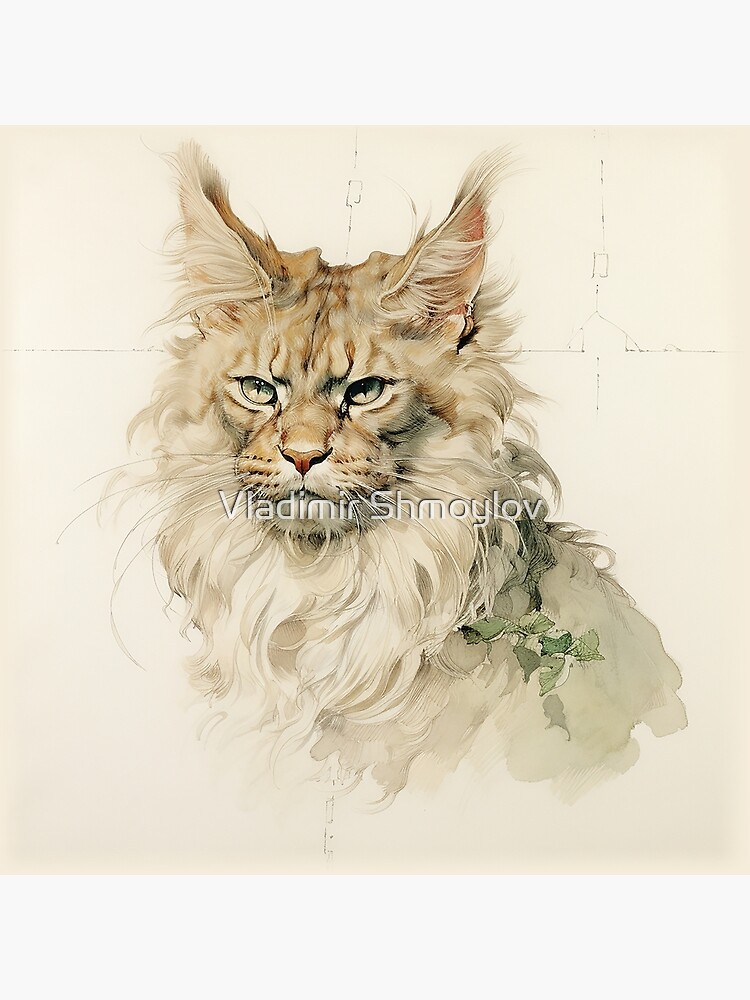The image is a detailed and striking drawing of a cat that bears strong similarities to a bobcat or even a mountain lion, largely due to its pointed ears featuring characteristic tufts of hair. The cat's face is a blend of features from both domestic and wild cats, with a broad and strong muzzle that houses long, white whiskers. The cat's fur is particularly noteworthy for its length and fluffiness, with a mix of orange, black, brown, and white colors. Its face exudes a mean and somewhat intimidating demeanor, akin to that of a lion or tiger, and it has piercing gray eyes. A green collar, resembling a string of leaves, adorns its neck. The body, partially visible below the mane, has shades of gray and green. The background is a very light pink, and prominently written across the middle of the image in white letters is the name "Vladimir Shmoilov," likely the artist.